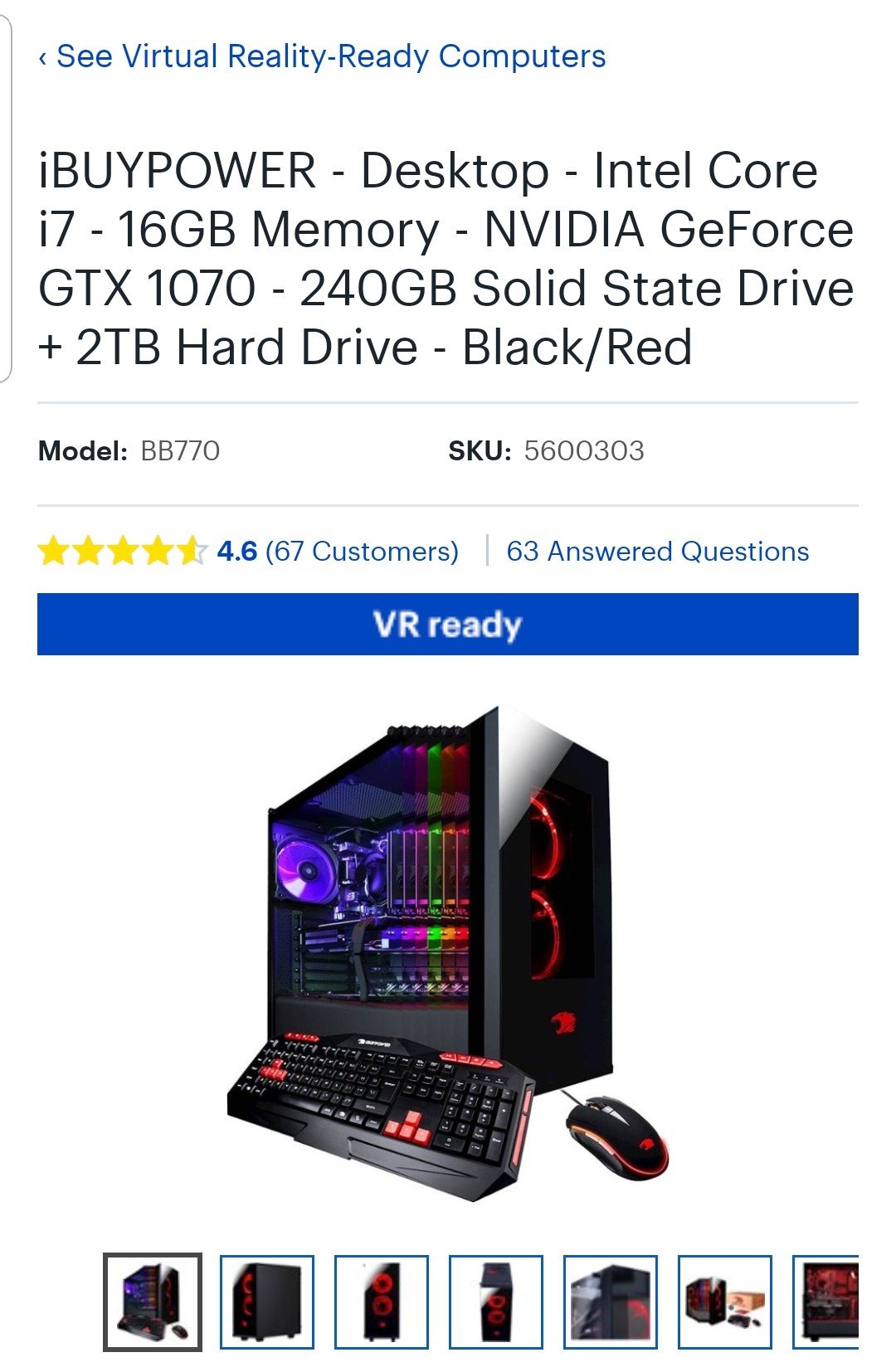This detailed caption describes a screenshot of a product listing on the BestBuy website:

The screenshot showcases a PC listing prominently displayed at the top of the BestBuy website. The title, written in bold blue, clickable text, reads "See Virtual Reality-Ready Computers," with a left-pointing arrow next to it. Below, in black text, it lists the PC's brand and specifications: "iBUYPOWER - Desktop - Intel Core i7 - 16GB Memory - NVIDIA GeForce GTX 1070 - 240GB Solid State Drive + 2TB Hard Drive - Black/Red." The brand "iBUYPOWER" is in all caps, except for the "i" and "a."

On the left-hand side, in bold black text, it says "Model," followed by "VB770." Underneath, another bold black text reads "SKU," with "5600303" in regular black text. The product has a rating of 4.6 out of 5 stars, based on 67 customer reviews, which is displayed in parentheses in blue text. To the right, it shows "60 Answered Questions."

Below the product details, a dark blue rectangle contains bold white text that reads "VR Ready," with "VR" capitalized. The PC case itself is black with red fans in the front and a purple fan in the back. Inside the case, cascading colors of purple, pink, red, and green illuminate the components. Accompanying the PC is a black keyboard with red keycaps on the WASD keys, arrow keys, and some keys at the top. The mouse also features a black design with red accents. The listing includes a panorama of images showcasing various angles of the computer case.